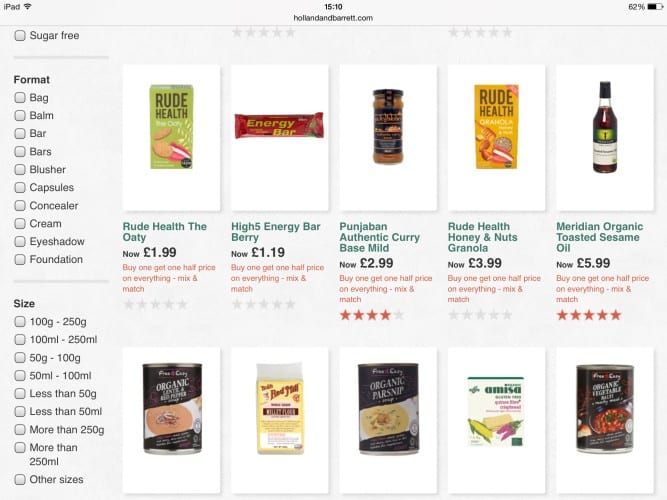Here is the cleaned-up and detailed descriptive caption for the image:

---

**Caption:**

A screenshot from an iPad displayed against a white backdrop. In the top-left corner, an "iPad" label, with a lowercase "i" followed by the word "pad," can be seen. To the right, the Wi-Fi signal strength icon appears in black. Centered across the top, the time "15:10" (3:10 PM) is displayed, beneath which the website "HollandandBarrett.com" is written in black. Next to the time, there is a battery icon, half-filled, showing "62%."

Further down on the left side, there is an empty gray box with the text "sugar-free" adjacent in black. Next to this, there are two sets of five gray outlined stars. 

Below this, there is a vertical drop-down menu in black text. At the top, "Format" appears in bold, followed by a list of single words — each paired with an empty gray box on the left: "Bag," "Balm," "Bar," "Bars," "Blusher," "Capsules," "Concealer," "Cream," "Eyeshadow," and "Foundation." A gray line separates this from a new section titled "Size" in bold. This section includes listings of size ranges next to gray boxes: "100G - 250G," "100ML - 250ML," "50G - 100G," "50ML - 100ML," "Less than 50G," "Less than 50ML," "More than 250G," "More than 250ML," and "Other sizes."

To the right of the drop-down menu, there are two rows of product images, each row containing five images. The first row includes:
1. A green box labeled "Rude Health," priced at £1.99, with a red "Buy one, get one half price on everything - mix and match" promotion and five gray stars underneath.
2. A red energy bar wrapper labeled "Energy Bar" in yellow, "High Five Energy Bar" in green, priced at £1.19, and the same promotional offer in red.
3. A glass jar with a black label and lid, labeled "Punjaban Authentic Curry Base Mild," priced at £2.99.
4. A yellow box labeled "Rude Health Honey and Nuts Granola," priced at £3.99.
5. A glass jar with a green label and black lid, labeled "Meridian Organic Toasted Sesame Oil," priced at £5.99.

The second row features:
1. A can with a reddish-colored label showing a white bowl containing brown soup.
2. A plastic jar with a yellow label and red writing.
3. A can labeled "Organic Parsnip," showing a white bowl with yellow soup.
4. A white box with green writing, featuring an image of corn and a purple fruit near the bottom.
5. A can with a purplish label, partially visible text reads "organic" in white.

---

This version organizes and clarifies the information, making it comprehensive and easy to follow.